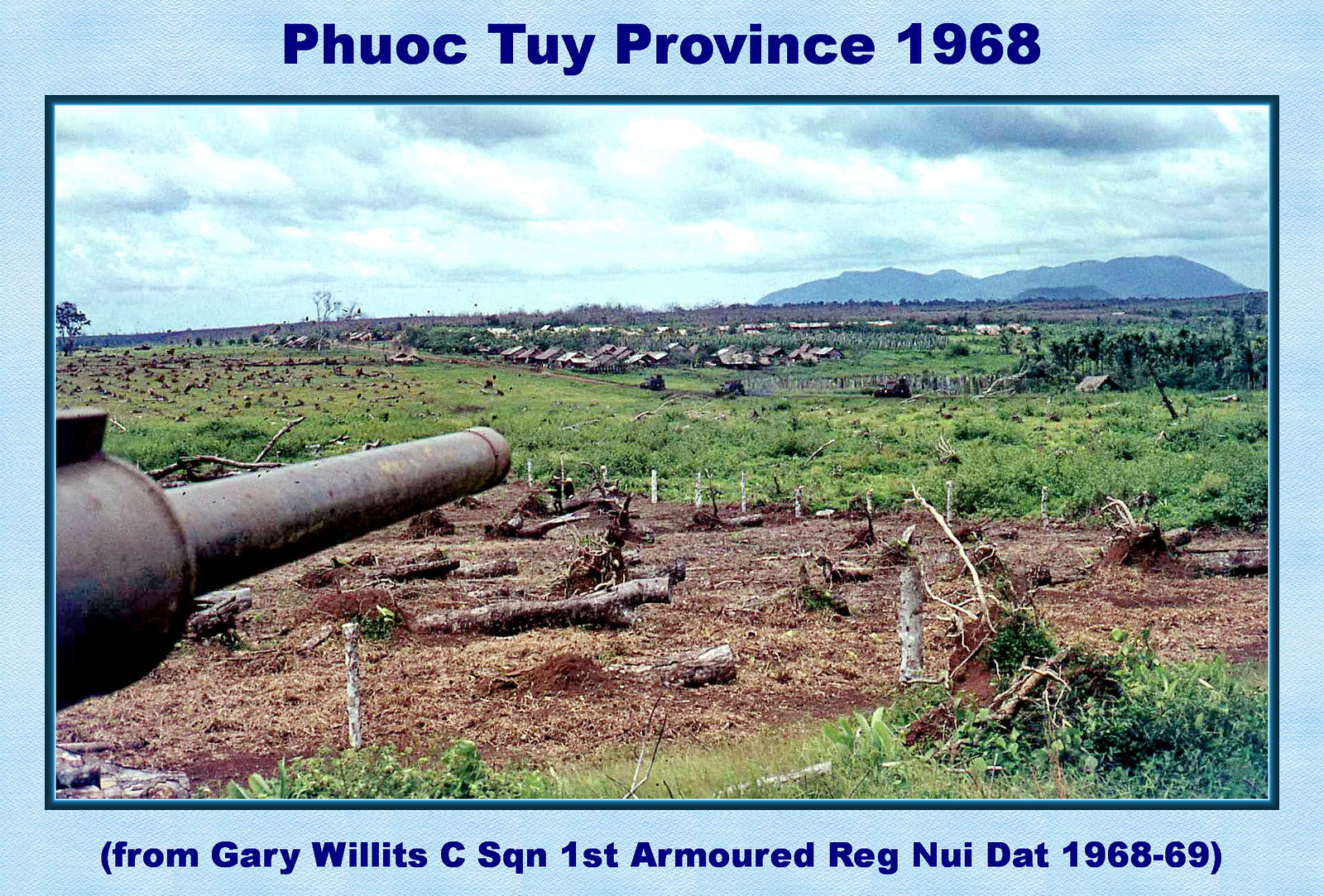This 1968 photograph captures the aftermath of a battlefield in Phuoc Tuy Province, Vietnam, bordered by a blue outline. The decimated ground is strewn with barren tree stumps, and a cannon or mortar with a long barrel is seen on the left-hand side of the image. In the background, green grass contrasts with a distant village of small huts, set against a mountain range. The sky above is dotted with both white and cobalt grey clouds, underlining the tranquil but somber scene of destruction. The caption above reads "Phuoc Tuy Province, 1968," while the bottom text states, "From Gary Willits, C-Squadron, 1st Armored Regiment, Nui Dat, 1968-69."